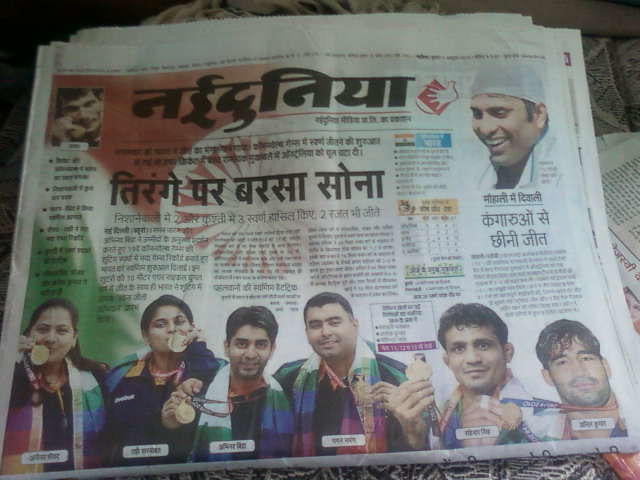The photograph features the front page of a newspaper from India, prominently displaying various elements in a foreign language. The newspaper is laid out on a table among other papers, folded in half to show the front page. Dominating the top portion is a bold black title, with smaller articles and detailed black text beneath. The upper left corner features a man pointing at the camera, while the upper right presents a man in a white hat, smiling and looking down.

Noteworthy imagery includes the iconic tricolor of the Indian flag with orange on top, white in the middle, and green at the bottom, and a circular sun pattern in the center. At the bottom of the page, six jubilant athletes, clad in colorful scarves, proudly display their gold medals. The women among them hold their medals close to their lips, kissing them, while the men present their accolades in front of them. All are beaming with pride, suggesting a recent triumph, possibly from the Olympics.